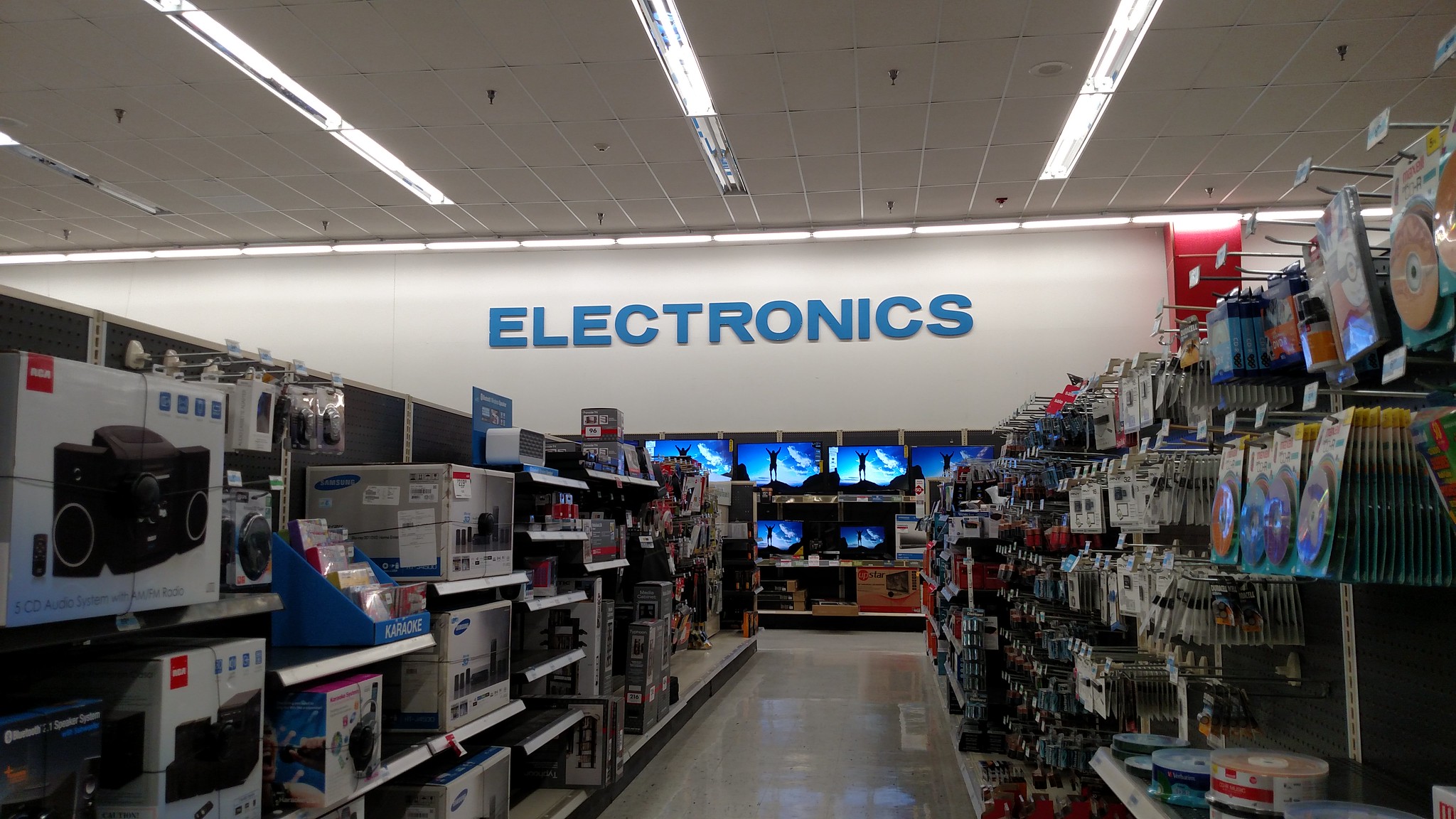The photograph captures the interior of a store's electronics department, characterized by an array of televisions, speakers, and related equipment. Dominating the white wall in the background is a prominent sign with large, blue letters that read "Electronics." This sign helps to clearly demarcate the section within the store. The photo is taken from an aisle viewpoint, revealing shelves lined with boxed speakers and various other pieces of electronic equipment. Further down the aisle, near the end where the electronics section sign is positioned, a variety of televisions are on display. These TVs are turned on and collectively showing an image featuring a person standing against a blue background. The overall scene captures the bustling, tech-filled environment of the store's electronics department.